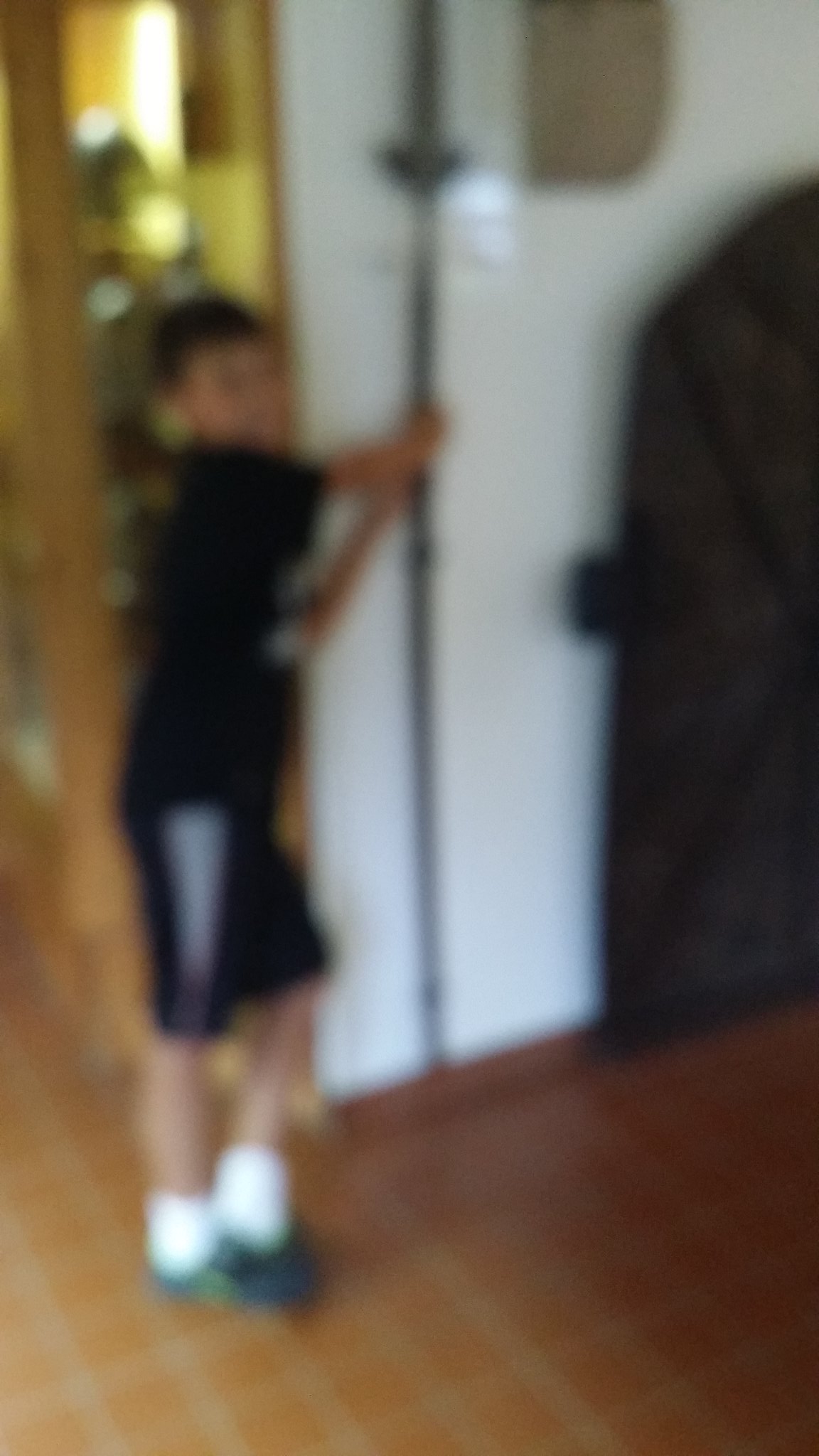A highly blurred image featuring a scene with various elements. At the bottom and towards the back, a white wall can be seen, and the floor is covered in brown tiles. On the left side of the image, a boy with short hair is present. He is wearing a black shirt, white socks, and black shoes. Despite the blur, he seems to be holding an object on the right side of the image, possibly resembling a sword. In the background, there is a light brownish hue, providing a slight illumination to the scene. The ground appears to have light-colored tiles mixed in with the brown ones. The character on the right also seems to be dressed in a black shirt.